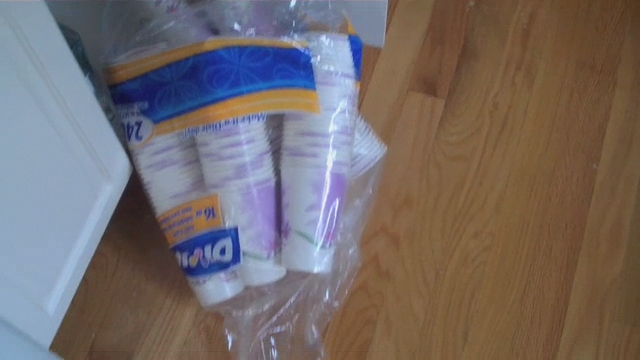The image is a slightly out-of-focus color snapshot, looking down on a light oak hardwood floor, likely in a kitchen. On the left side, the bottom row of white base cabinets is visible, with one cabinet door in clear view. Dominating the scene is a large, clear plastic industrial-sized bag of Dixie cups, lying upside down on the floor. The bag prominently displays the Dixie brand on a blue banner background and indicates it contains 240 white 16-ounce cups. Each cup is stacked inside another and features a purple splash design. The scene’s central focus is the expansive bag of cups, although the slightly blurry quality makes finer details less discernible.